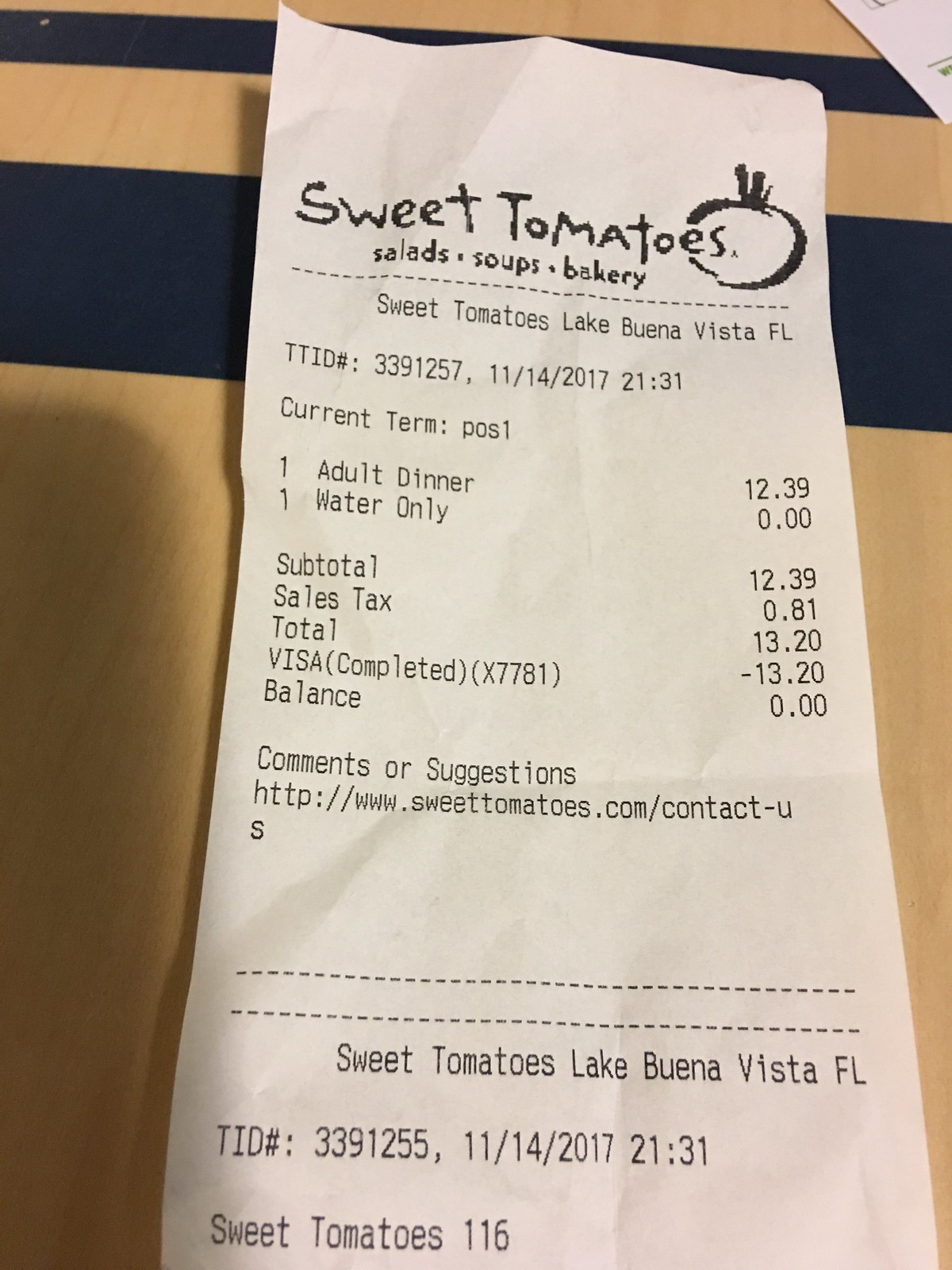This is a color portrait photograph of a receipt positioned vertically against a light brown surface. The receipt is white with clearly legible black text. The background features a wide navy blue stripe near the top, with a thinner dark blue stripe above it. The receipt is from a restaurant named "Sweet Tomatoes," located in Lake Buena Vista, Florida, and lists offerings such as salads, soups, and bakery items. The total amount on the receipt is $13.20, which was paid using a Visa card. The date of the transaction is November 14, 2017.